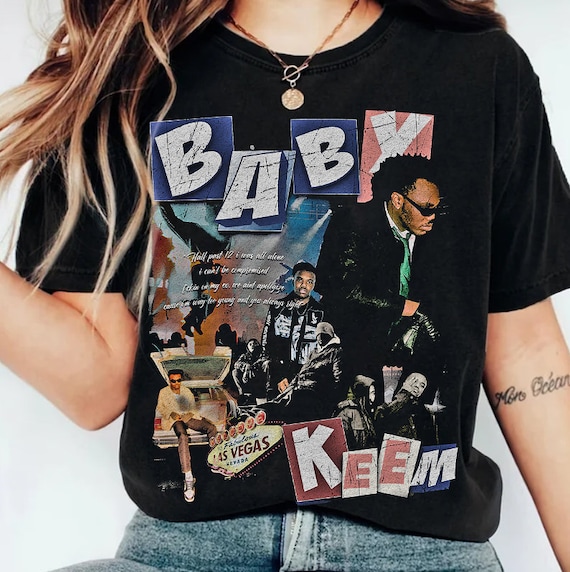The image features the torso of a long-haired individual, likely a woman, with straight, blondish hair and a visible tattoo on her left forearm. The central focus is her black t-shirt, which prominently displays the text "Baby Keem" in two parts, with "Baby" at the top and "Keem" at the bottom. This shirt includes various images of a black gentleman in different poses, arranged in a collage, along with a depiction of the "Welcome to Fabulous Las Vegas Nevada" sign, suggesting the person on the shirt may be an entertainer or musician. The woman also wears a necklace and gray bottoms. The background is stark white, giving the impression of a fashion shoot.